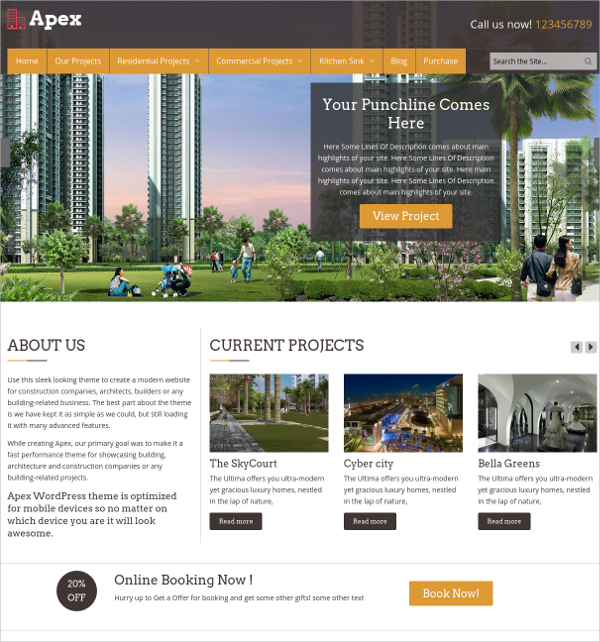The webpage features a sleek design optimized for construction companies, architects, builders, and other building-related businesses. At the top of the page, a dark banner is showcased, prominently displaying "APEX" in white lettering alongside a red line drawing of two buildings in the top-left corner. In the top-right corner, visitors are prompted to “Call Us Now: 1-2-3-4-5-6-7-8-9.” Below this, an orange navigation menu is neatly arranged with options: Home, Our Products, Residential Projects, Commercial Projects, Kitchen Sink, Blog, and Purchase. To the right of the menu, there's a gray search bar labeled "Search the Site."

The main section of the page displays a vibrant photograph of numerous tall buildings with a lush, park-like area in the foreground. The scene depicts people sitting on the grass and walking around among numerous trees, encapsulating a blend of urban and natural environments. Overlaid on the image is a gray pop-up window containing placeholder text: "Your punchline comes here. Here are some lines of description about the main highlights of your site," followed by an orange button labeled "View Project."

At the bottom left of the page, it reads, “About Us: Use this sleek-looking theme to create a modern website for construction companies, architects, builders, or any building-related business. The best part about the theme is we have kept it as simple as we could, but still loaded it with many advanced features. While creating Apex, our primary goal was to make it a fast performance theme for showcasing building, architecture and construction companies or any building-related projects. Apex WordPress theme is optimized for mobile devices, so no matter on which device you are, it will look awesome.”

To the right, under the "Current Projects" section, three ongoing projects are highlighted:

1. **SkyCourt**: "The Ultima offers you ultra-modern yet gracious luxury homes nestled in the lap of nature."
2. **Cyber City**: The same description as SkyCourt.
3. **Bella Greens**: The same description as SkyCourt and Cyber City.

Accompanying these projects is a promotional message announcing an ongoing offer: “Online booking now, 20% off, hurry up to get an offer for booking and get some other gifts,” concluded by an orange “Book Now” button for immediate action.